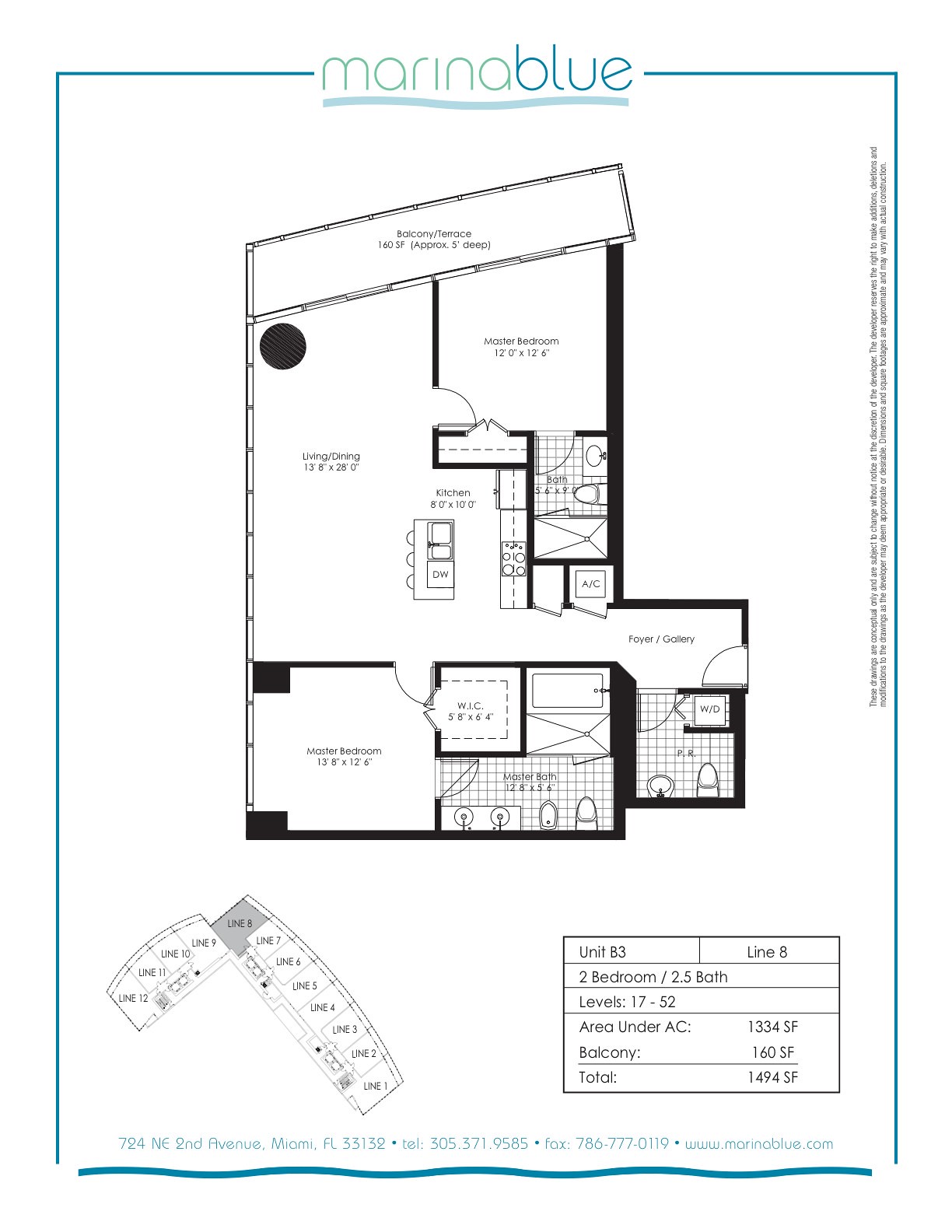A detailed black and white schematic blueprint of an apartment is displayed against a white background, illustrating an L-shaped layout reminiscent of a boxy Christmas stocking. The intricate top-down design meticulously marks the placement of doorways, bedrooms, and bathrooms across the unit. In the bottom right corner, a labeled box provides specific details: the unit is identified as Unit 83, Line 8 and includes two bedrooms and 2.5 bathrooms. It serves occupants from levels 17 through 52. The total area of the apartment is 1,494 square feet, with 1,334 square feet under air conditioning, and a balcony area totaling 160 square feet. This professionally drafted sketch offers a clear and precise visualization of the apartment's structure and dimensions.